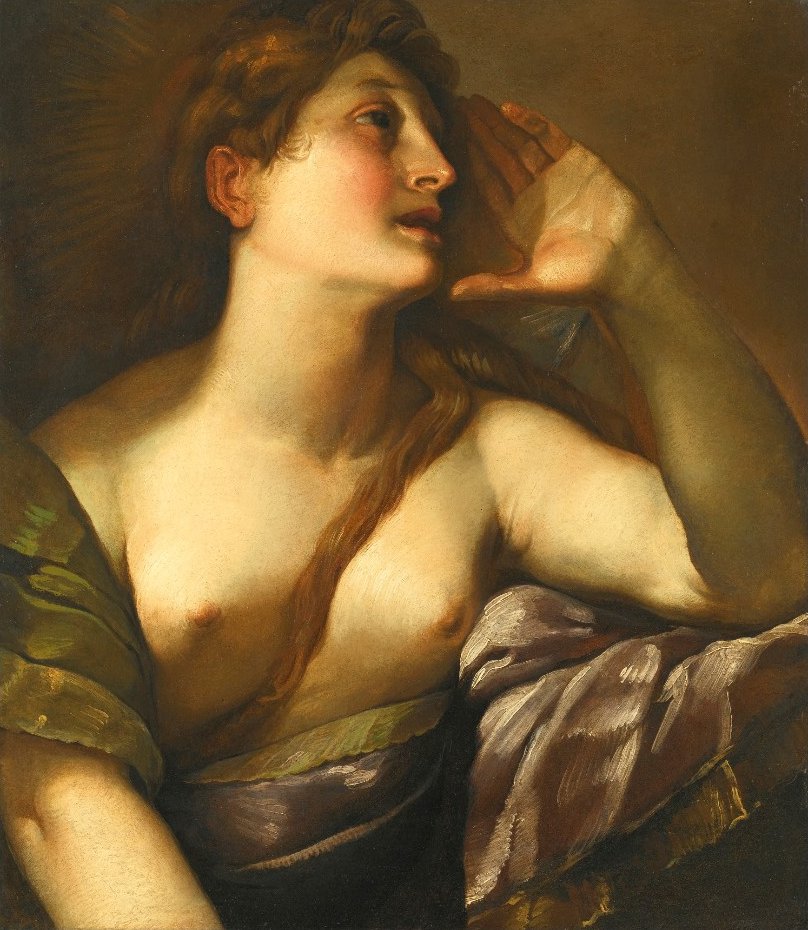This painting, rendered in warm tones of yellows, greens, and golds, depicts a bare-chested woman with reddish-brown, almost reddish-golden hair that flows over her back and drapes across her left shoulder, falling between her breasts down to her waist. She is facing to the right, her face partially in profile, with her right ear visible. Her expression is one of notable distress, with wide, pleading eyes and a partially open mouth, suggesting she's in some sort of pain or mental anguish. Her left hand is raised to her face, forming a V shape, with her thumb near her chin and her fingers extending up towards her forehead. A piece of green fabric drapes over her right shoulder, while her left arm rests on a pinkish-purple fabric. Additionally, she is wrapped in a robe that appears predominately green and gray with hints of purple, secured with a yellow band at her waist. The overall scene evokes a dramatic, emotional ambiance focused on the woman's palpable suffering.